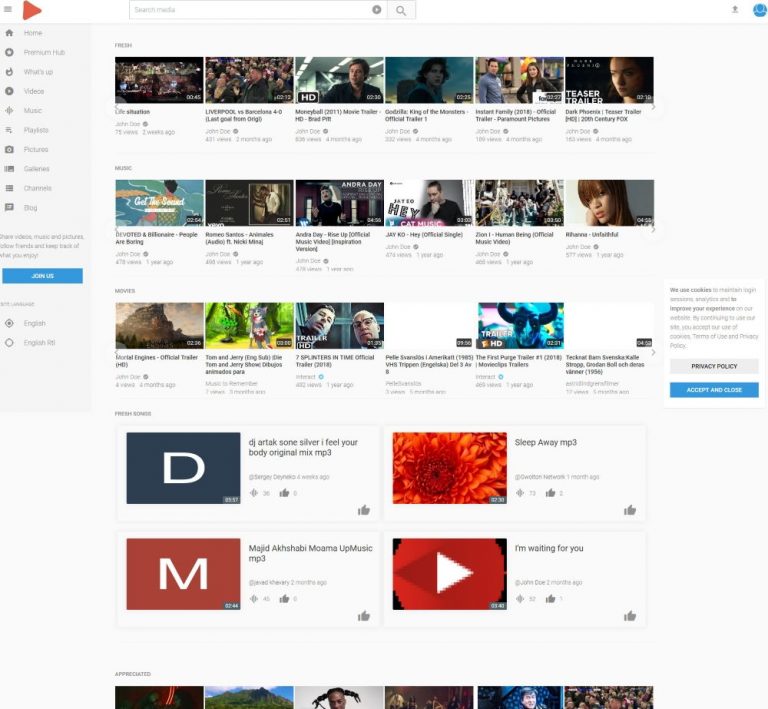This image features a webpage that resembles a YouTube-like platform. In the upper left-hand corner, there is a distinctive, filled red arrow pointing to the right. Adjacent to the arrow is a navigation menu listing 10 clickable options: Home, Something Hub, What's Up, Video, Music, Playlists, Pictures, General, Channel, and Blog. Each option has a small, barely visible icon next to it. 

The main body of the page is organized into rows of video thumbnails. The top section displays three rows, each containing six video thumbnails, amounting to 18 video previews in total. Below these rows, there is a distinct section featuring four prominently displayed videos, likely highlighted or recommended content. Following this featured section, the layout continues with additional rows each containing six video thumbnails, mirroring the arrangement seen in the initial rows.